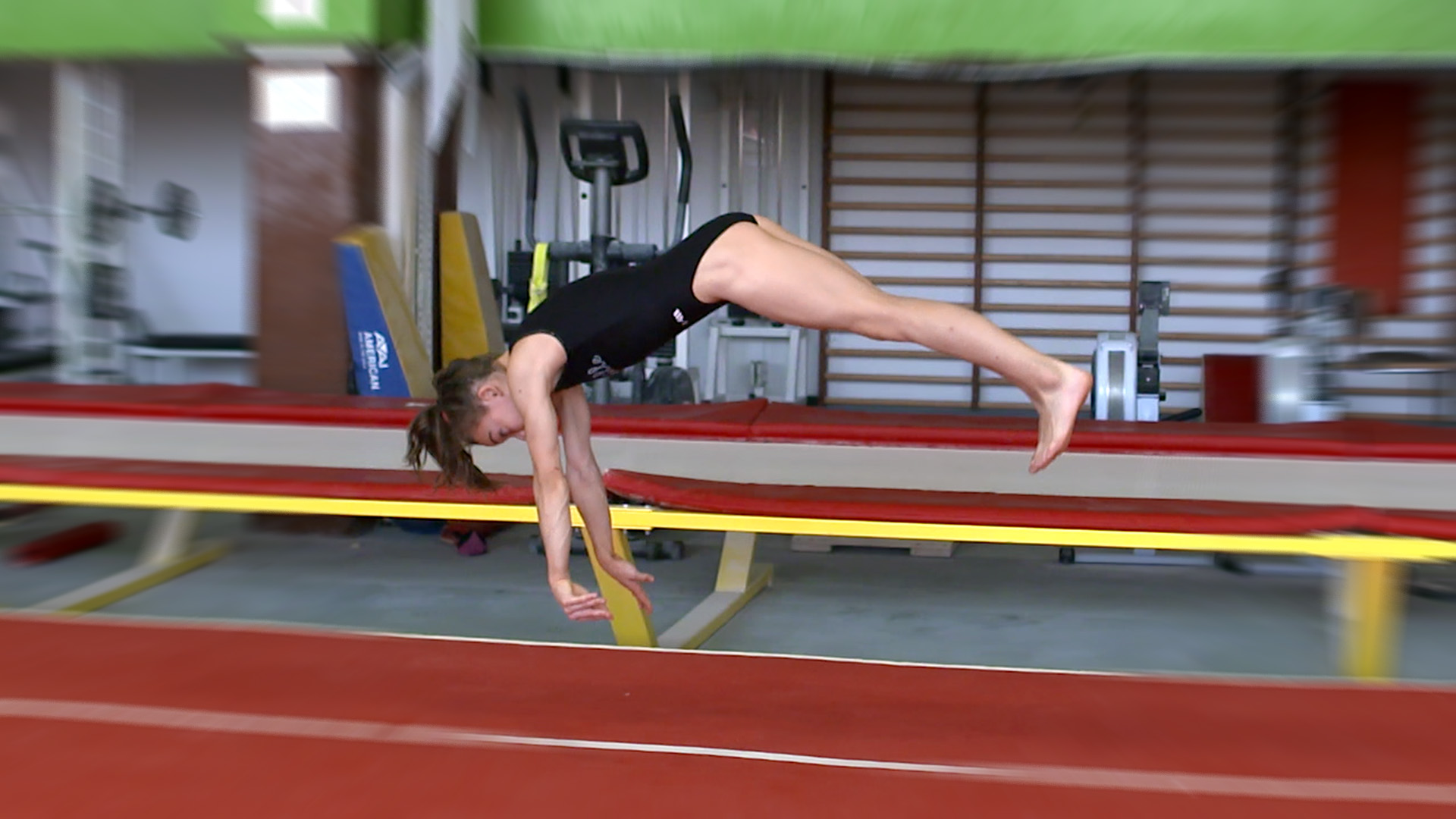In this detailed photograph, a young female gymnast, dressed in a tight black one-piece gymnastic suit, is captured mid-flip in a dynamic, airborne pose. She has brown hair tied in a ponytail, accentuating her focused expression. Her body is positioned with her head pointing down towards the lower left corner, her feet towards the right lower corner, and her arms stretched out directly downwards, as if she's diving gracefully toward the ground.

The setting appears to be a comprehensive sports facility. In the background, there is a red running track field, contrasting with green surface areas, suggesting a multi-use training ground. Additionally, one can discern gym equipment such as a stair climber, a bicycle machine with handlebars, and a weight lifting set, indicating a well-equipped athletic environment. The gymnasium walls and a door frame further emphasize the training atmosphere. The image is sharply focused on the gymnast, while the peripheral area remains slightly out of focus, drawing the viewer's attention to her impressive athletic form suspended in the air.